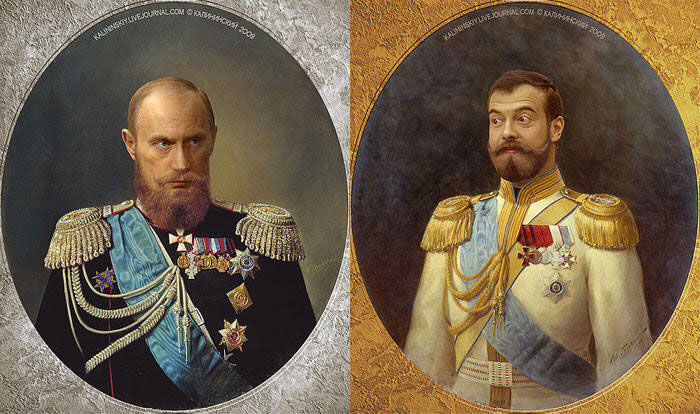This detailed image features two high-ranking military officials, each prominently displayed in separate photographs, possibly on cards. Both men are adorned in their full regalia, showcasing an array of badges, medals, and tassels reflecting their decorated status. The man on the left has less hair and appears more decorated, while the man on the right has more hair. Both individuals sport beards and mustaches, adding to their distinguished appearance. They are positioned with the man on the left looking towards the center and the man on the right also facing towards the center, though their gazes do not meet.

The background of the image reveals a blend of colors including shades of gray, tan, blue, black, red, orange, yellow, silver, gold, cream, purple, and various hues associated with the medals and uniforms. There's also text arched above each photo, though it's too small to decipher clearly, with only the year 2009 being somewhat legible. The overall setting and style suggest that these are older images of generals, encapsulated in a visually creative presentation that could be a painting or a detailed drawing, embodying an air of historical significance.